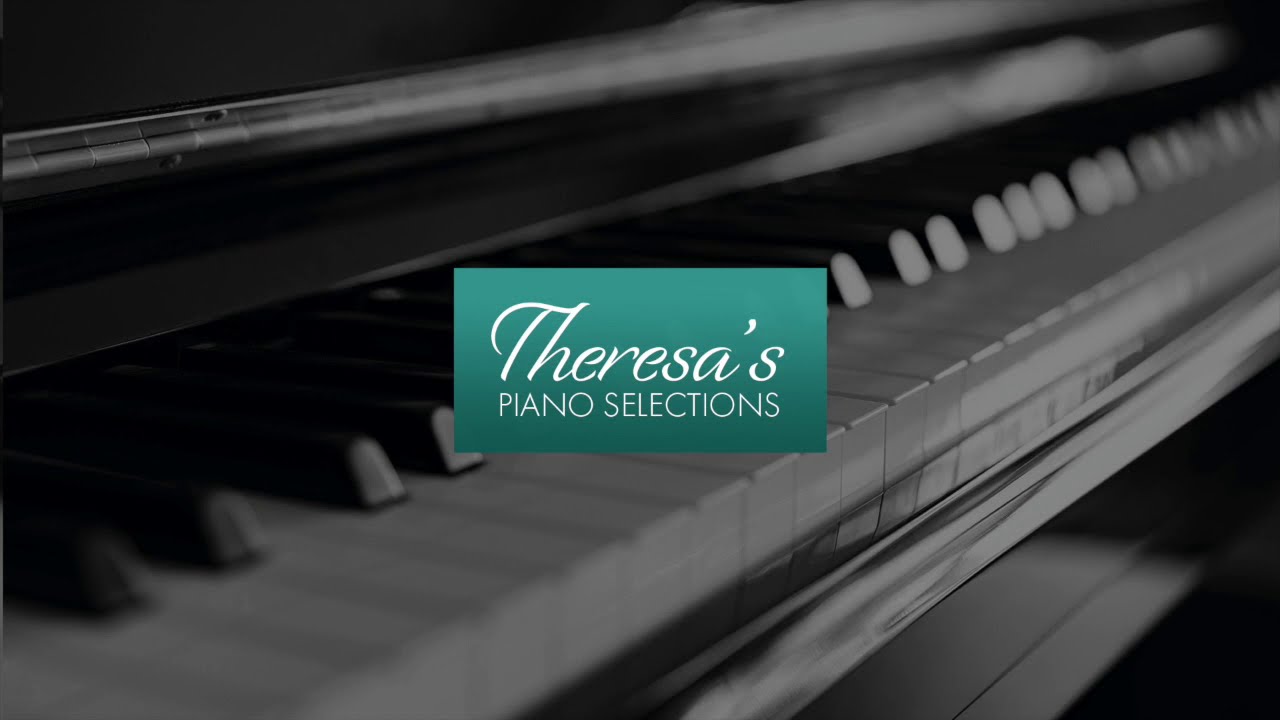In the monochromatic image, a dark black piano extends diagonally from the bottom left to the top right, with its array of black and white keys prominently featured. This grand piano, likely crafted from dark wood, is complemented by a matching black band chair situated beneath it. Dominating the center of the image is a green rectangle bearing the inscription "Teresa's Piano Selections." The text "Teresa's" is elegantly written in a cursive white font, while "Piano Selections" is displayed in all uppercase letters, also in white. The image has a graphic, shadowy quality, making the keys and background appear in varying shades of grey and black, and suggesting it could be a cover for a CD, record, or a header for a blog or web page, evoking a sophisticated, vintage atmosphere.